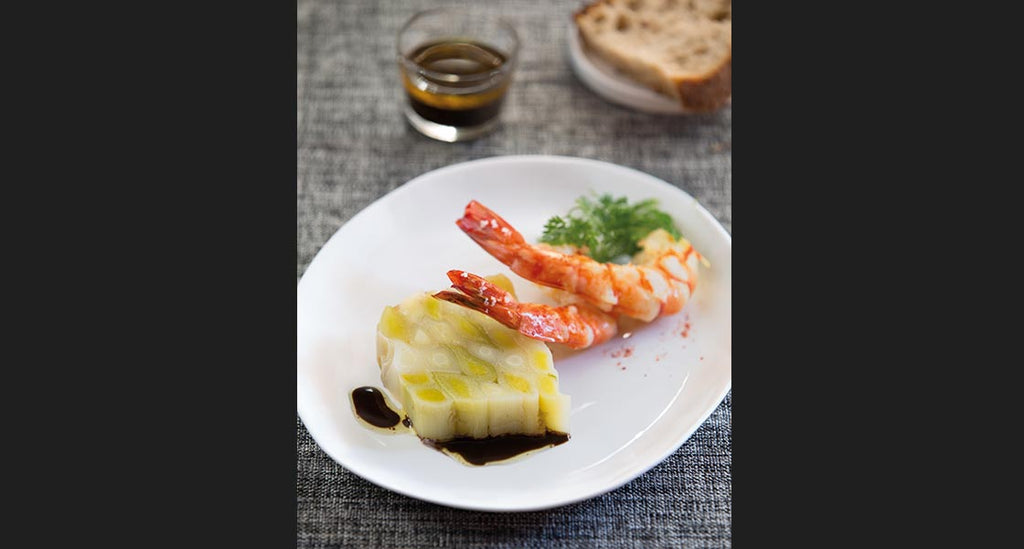The image is a close-up color photograph of a carefully arranged plate of hors d'oeuvres, set on a dark gray, heathered tablecloth. The focus is on a round, white plate positioned prominently in the center of the horizontal rectangular frame, flanked by vertical black stripes on either side. The dish features two large, cooked shrimp with orange and white hues, their tails still attached, located to the right of the plate. Garnishing the shrimp is a small sprig of parsley, adding a touch of green. On the bottom left of the plate lies a square piece of food in varying shades of yellow, possibly a slice of pickled artichoke or another type of seafood, detailed with ridges and drizzled with a bit of black sauce. Past the main plate, slightly out of focus, is a clear glass container holding a brown liquid, possibly a sauce or more olive oil, and a smaller plate presenting a slice of brown bread. The composition and intricate details suggest a sophisticated culinary presentation.